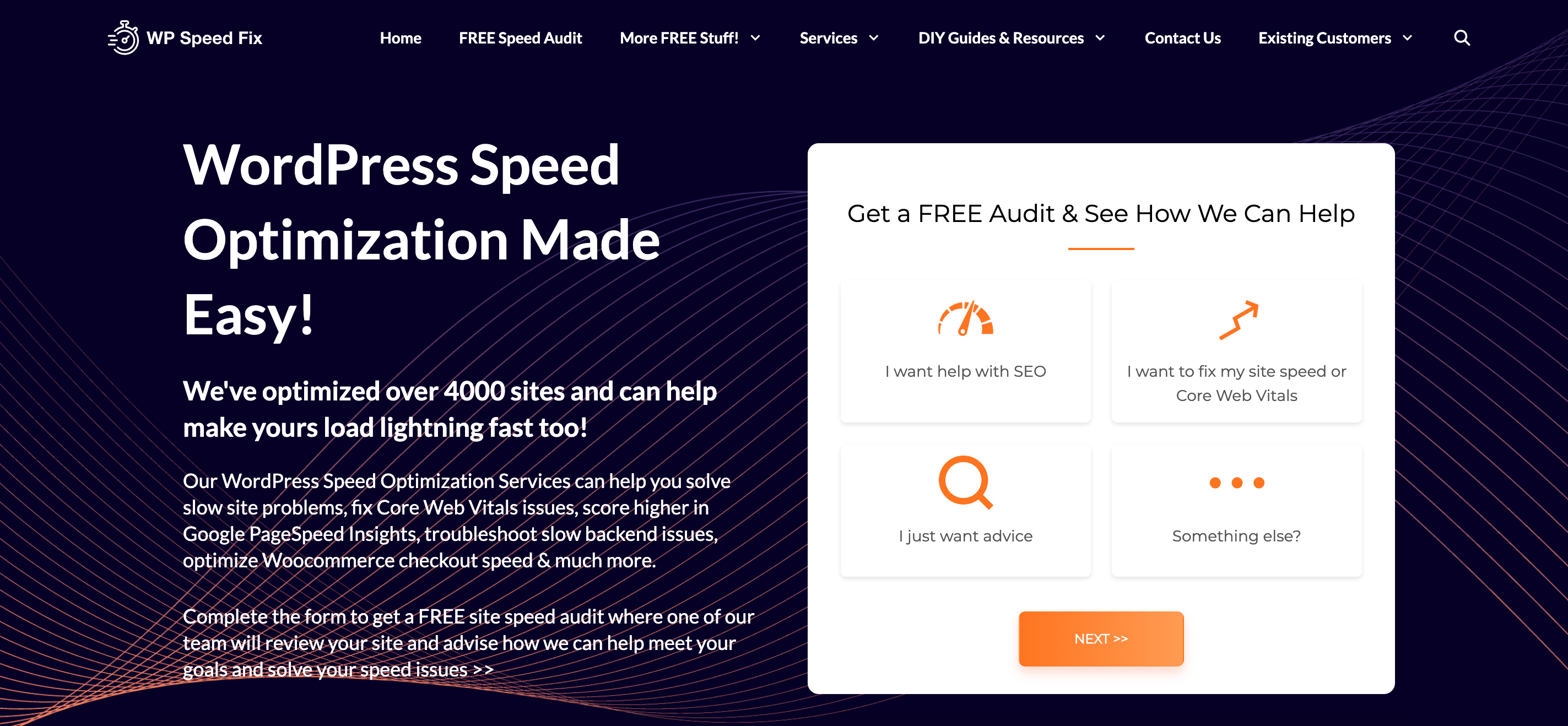### Website Landing Page for WP Speed Fix

**Header:**
- Background: Navy blue with dynamic red wavy lines.
- Logo: "WP Speed Fix" in bold white letters at the top.
- Navigation Bar (White Text): 
  - Home 
  - Free Speed Audit
  - More Free Stuff
  - Services
  - DIY Guides and Resources
  - Contact Us
  - Existing Customers
- Search Icon: Magnifying glass for site search functionality.

**Main Content:**
- Slogan (White Text, Left-Aligned): "WordPress Speed Optimization Made Easy"
  - Subtext: "We’ve optimized over 4,000 sites and can help make your load lightning fast too. Our WordPress Speed Optimization Service can help you solve slow site problems, fix core web vital issues, score higher in Google PageSpeed Insights, troubleshoot slow backend issues, optimize WooCommerce checkout speed, and much more."
- Call to Action (White Box, Centered): 
  - Text: "Get a Free Speed Audit and see how we can help"
  - Form Prompt: "Complete the form to get a free speed audit where one of our team will review your site and advise how we can help meet your goals and solve your speed issues."

**Visual & Usability Details:**
- Consistent color scheme with navy blue background and white text for excellent readability.
- Red wavy lines add a modern and dynamic feel.
- Clear and concise information hierarchy.
- Easily accessible navigation menu for a better user experience.
- Prominent call-to-action inviting users to engage with the service.

**Summary:**
The landing page for WP Speed Fix showcases a professionally designed website with a clear focus on WordPress speed optimization services. It adeptly combines aesthetic elements like the navy blue background and red wavy lines with functional aspects such as an intuitive navigation menu and detailed service descriptions for an engaging and informative user experience.